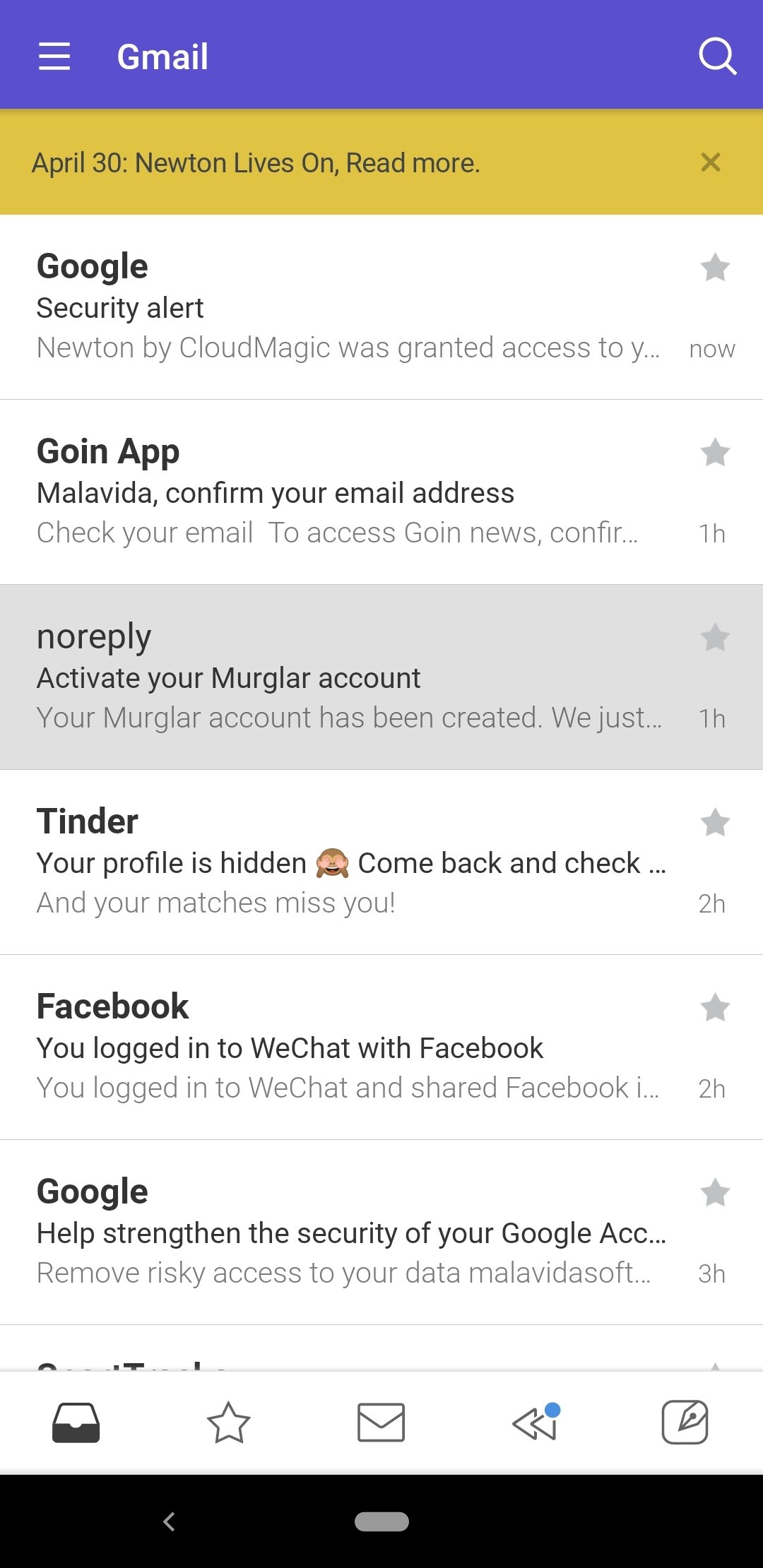**Header Section:**
The top header has a dark violet background. On the left, there are three white horizontal lines indicating a collapsible submenu. To the right of these lines, "Gmail" is prominently displayed in bold white font. Far right, there is a white magnifying glass icon representing the search function.

**Secondary Header:**
Below the top header, there is a secondary header with a gold background. In black text, it reads: "April 30: Newton lives on. Read more."

**Email Listings:**
Below the headers, the background transitions to white, showcasing individual email listings, each separated by a thin gray line.

1. **First Email:**
   - **Sender:** Google (in bold black font)
   - **Subject:** Security alert (in smaller, non-bold black font)
   - **Preview:** "Newton by Cloud Magic was granted access to Y..." (in gray text)
   - **Timestamp:** "now" (in small gray text at the far right)
   - **Star Indicator:** A gray star icon is located at the top right.

2. **Second Email:**
   - **Sender:** G-O-I-N app (in bold black font)
   - **Subject:** Malavita, confirm your email address (in smaller, non-bold black font)
   - **Preview:** "Check your email to access go in news, confirm..." (in gray text, truncated with ellipsis)
   - **Timestamp:** "1H" (indicating the email was sent one hour ago, in small gray text at the far right)
   - **Star Indicator:** A gray star icon is located at the top right.

3. **Selected Email:**
   - **Background:** The email is highlighted with a light gray background, indicating it is currently selected.
   - **Sender:** No-reply (in bold black font)
   - **Subject:** Activate your Murgler Account (in smaller, non-bold black font)